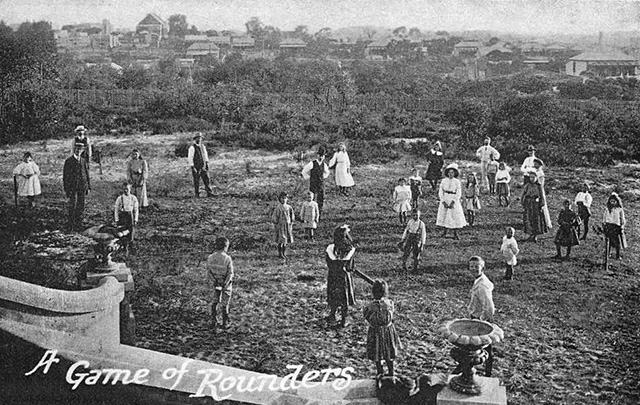This black and white overhead photograph, likely from the 1920s, captures a diverse group of people preparing for a game of rounders in a spacious, open field. The image, which is wider than it is tall, features individuals both facing and turning away from the camera, spaced approximately six feet apart. The men are dressed in suits or vests over white button-up shirts with slacks, while the women wear long-sleeved, shin-length white dresses, often accentuated with a waist belt. Prominently in the foreground, there is a stone wall, a felt birdbath, and a stone flower pot. White text in the lower left-hand corner reads "A game of rounders," indicating their activity. The background is filled with a view of residential buildings and a small forest, providing a sense of a serene suburban setting bustling with anticipation for the game.